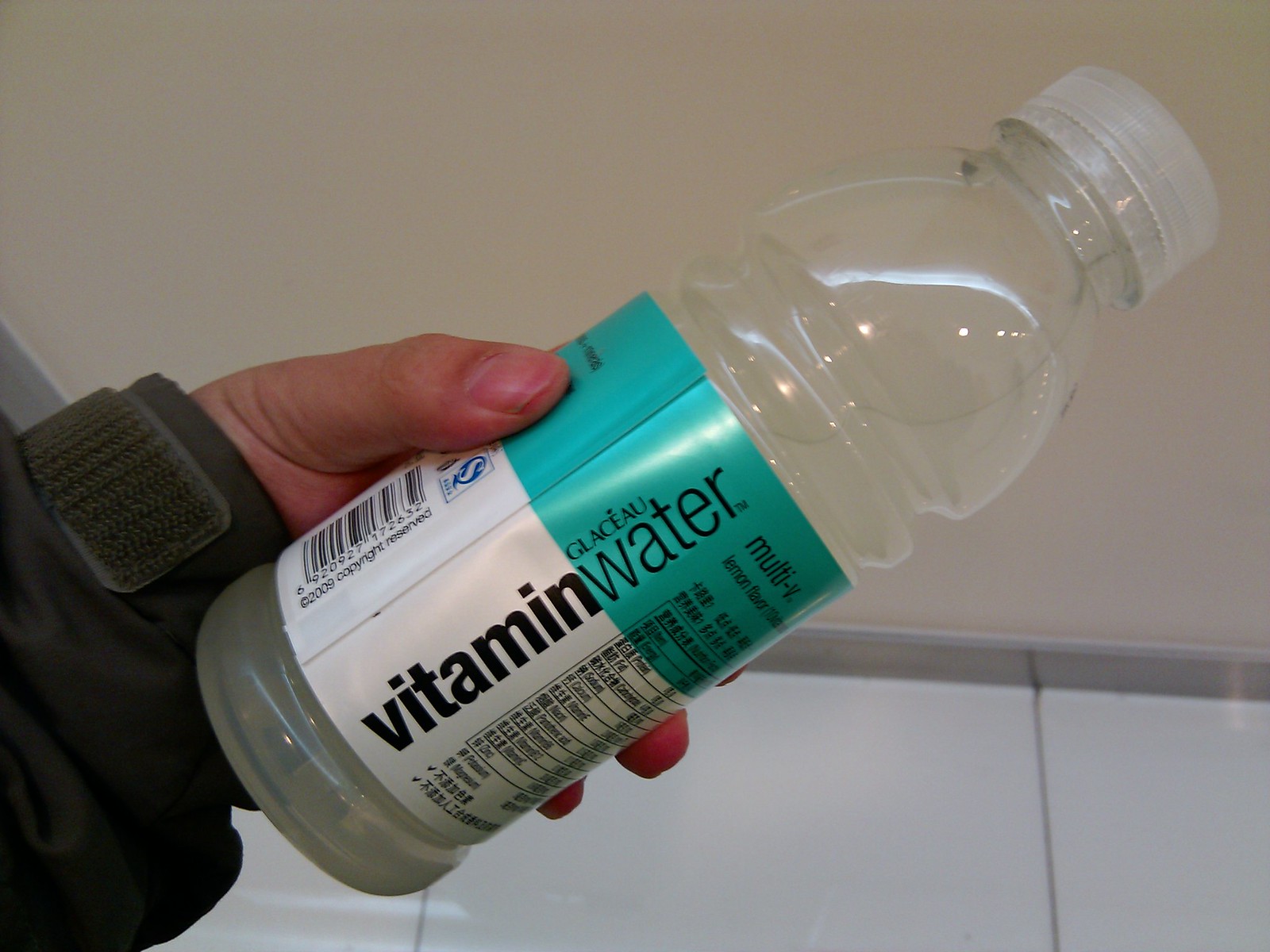In this image, a close-up shot showcases a hand holding a bottle of Vitamin Water. The hand appears from the bottom left, partially covered by a dark gray coat with a visible velcro strap near the wrist. The thumb rests on top of the bottle while the other fingers grip it from below, ensuring a secure hold. The Vitamin Water bottle is made of clear plastic, indicating that it is full, with a noticeable amount of liquid visible near the top.

The bottle features a label with a gradient design, transitioning from white at the bottom to turquoise blue at the top. The prominent text "Vitamin Water" is clearly legible, along with the term "multi-V" and a series of black labels on the right side of the label. Additionally, a black barcode is visible on the opposite side. 

The background includes a light gray floor and a tan-colored wall, providing a neutral setting that emphasizes the focus on the bottle and the hand holding it.